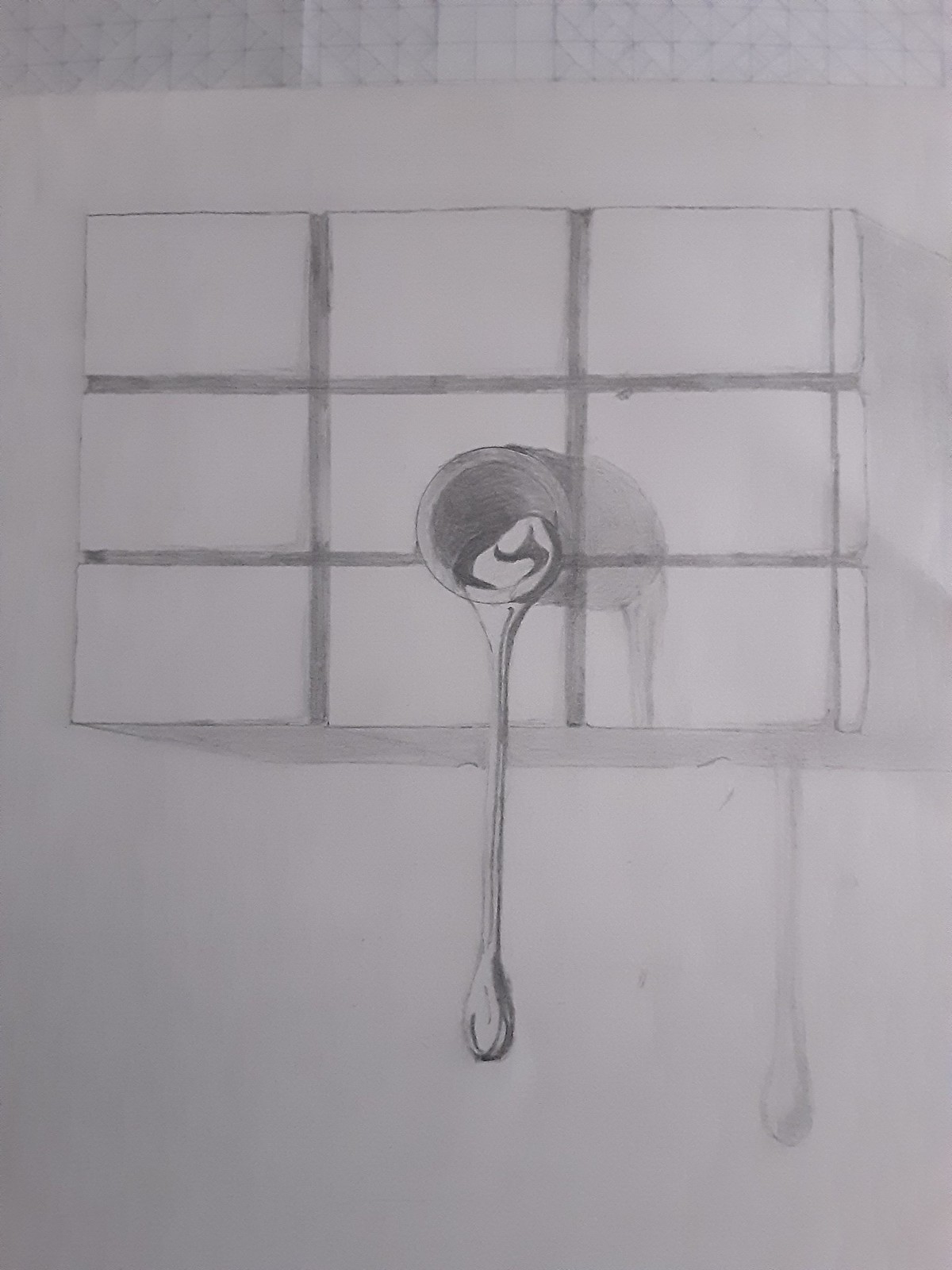This grayscale artwork, possibly a painting or drawing, is set against a textured, tile-like white surface. Dominating the composition is a rectangular object divided into nine smaller sections, each meticulously detailed to emphasize depth. Resting atop this object is a spoon filled with an unidentified liquid. The positioning of the spoon creates an intriguing interplay of shadows and reflections: its shadow extends to the right, falling over the rectangular object, while a reflection of its handle can be seen further to the right on the tiled surface below. The artist employs shading techniques to enhance the three-dimensionality of both the sections of the rectangle and the spoon, achieving a highly realistic yet distinctly illustrative effect.